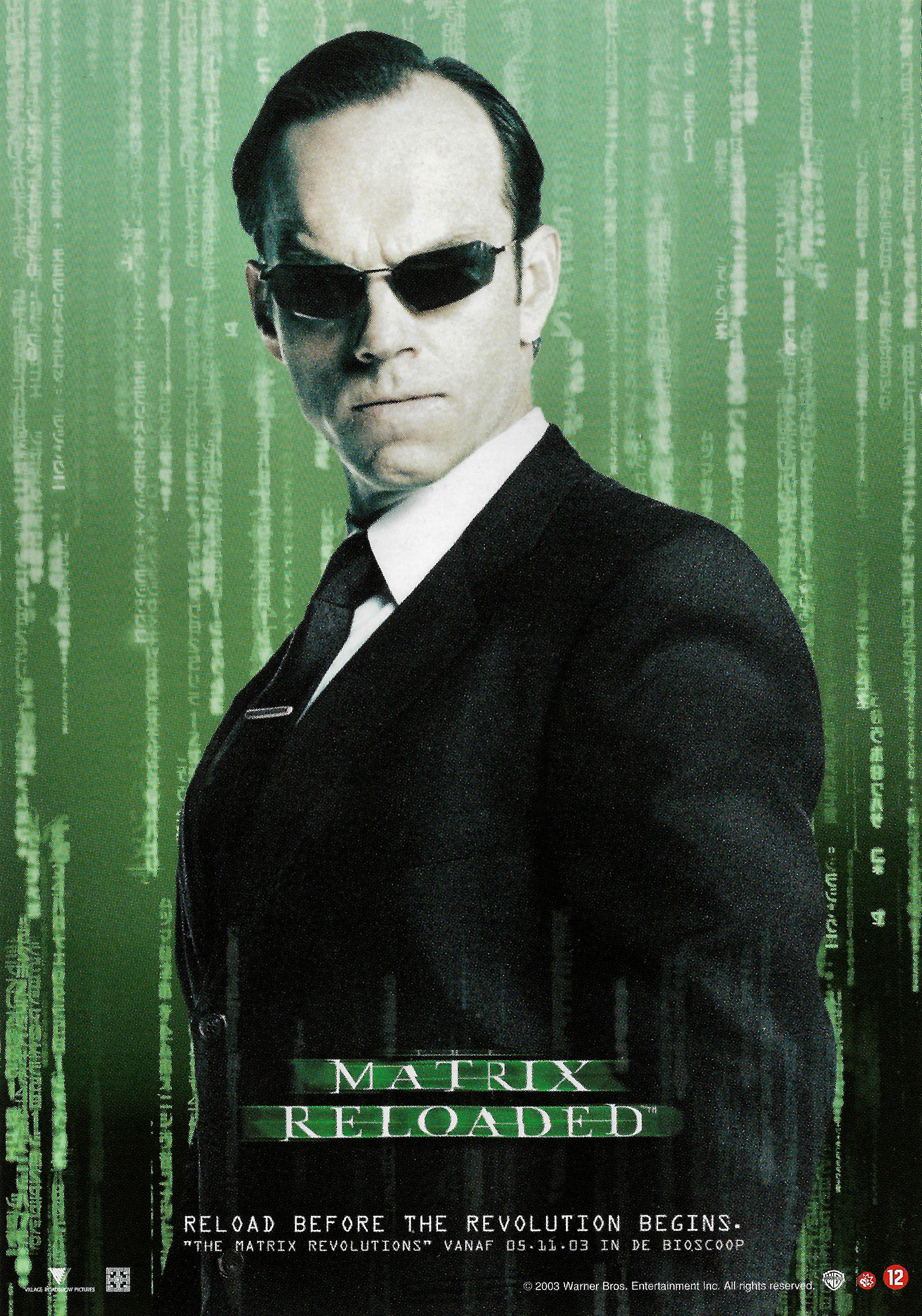The image is a promotional picture for "The Matrix Reloaded," featuring a professional movie scene setup. The man in the image has light skin and slicked-back hair, and he is wearing reflective black rimless sunglasses. He exudes a professional demeanor, wearing a black suit with a white button-up shirt and a black tie held in place by a silver and black tie clip. His face is facing forward, and he is raising an eyebrow, mugging for the camera. The backdrop consists of green and white computer code cascading from the top to the bottom, underscoring the film's iconic digital aesthetic. The code is not readable due to its small size. A green filter overlays the image, adding a slight green tinge to the man and blending with the gradient background that transitions from black at the bottom to light green at the top. The promotional text reads "The Matrix Reloaded: Reload Before the Revolution Begins," hinting at the connection to the subsequent movie, "The Matrix Revolutions." The only colors present in the image are black, white, gray, and varying shades of green, emphasizing the monochromatic and futuristic style synonymous with the "Matrix" series.